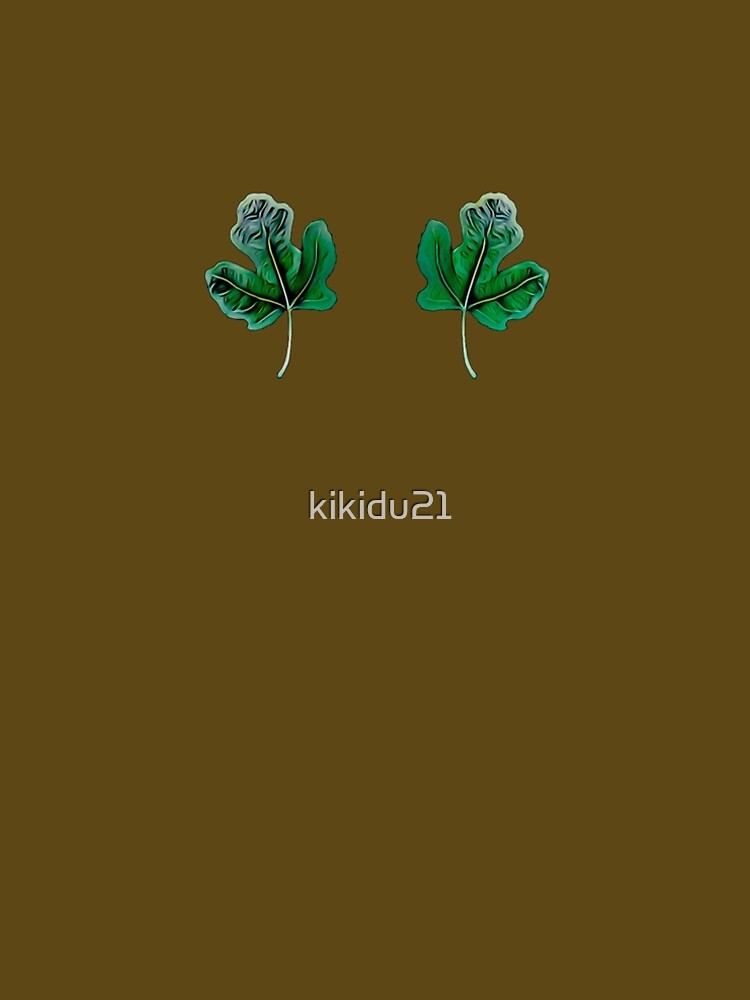The image is a vertically-oriented rectangle with the proportions of a standard US paper. It has a dark, muddy brown background. Positioned near the center are two very small, intricately detailed green leaves, each with three distinct sections and a curved stem that extends outward from the center. The white stems and veins are highlighted, and the center leaf of each pair has a small flowery part at its tip with some lighter, teal shading and black squiggly lines for added depth and texture. Underneath the leaves, in a clean, cream-colored font, is the text "Kikidu 21." The word "Kikidu" is in lowercase, while the "21" is in a larger font size, standing out against the minimalist background.